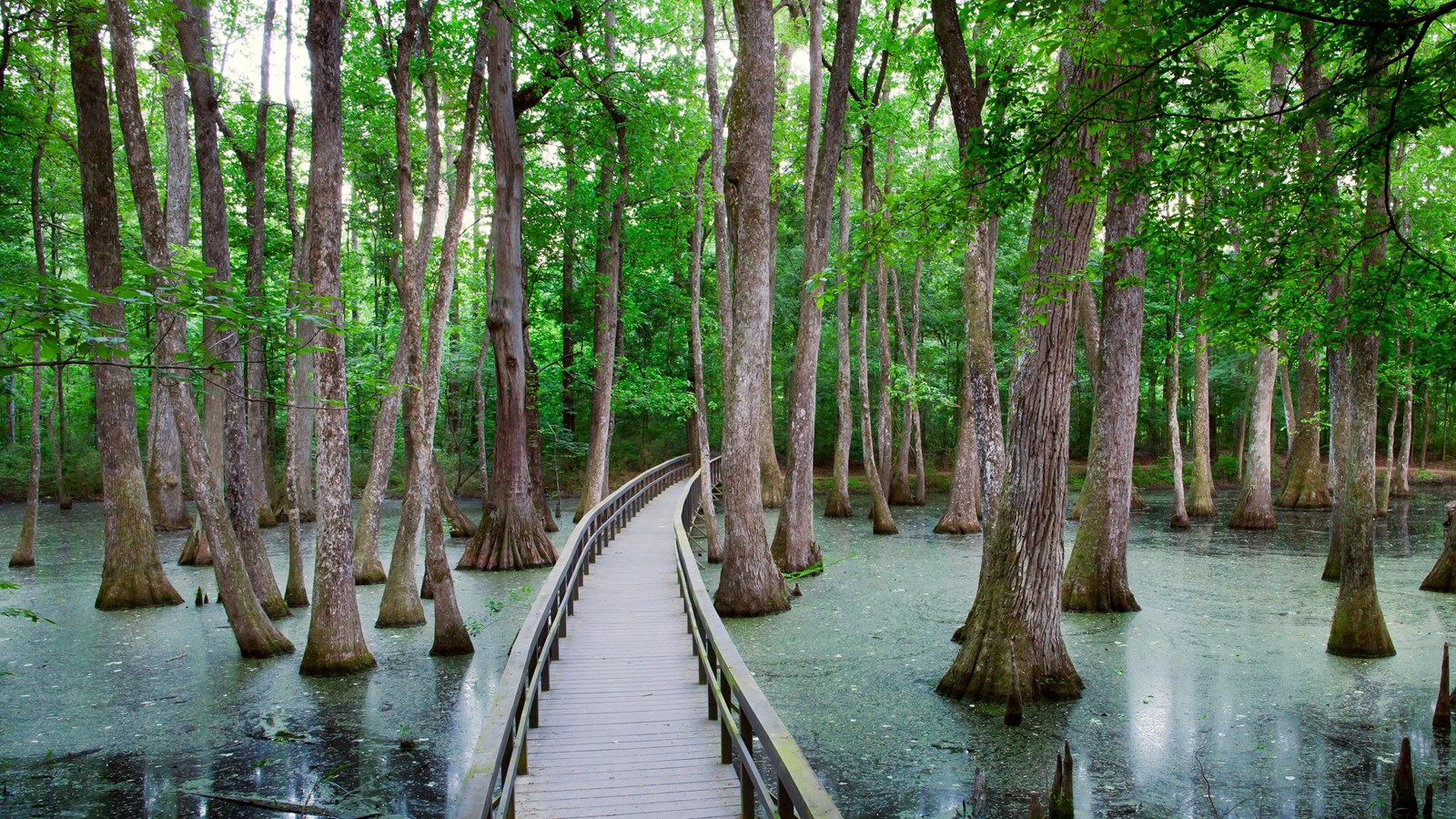In this detailed and evocative image, a grey metal bridge resembling a staircase stretches across a murky swamp. The bridge, covered in green pollen and leaves, has protective railings and is visually emphasized by layered steps. The surrounding swamp waters, dark and covered with greenish pollen, are flanked by tall, brown-barked trees with curved trunks and lush green foliage. Moss envelops the base of these trees, enhancing the sense of an undisturbed natural setting. The sky above is mostly white, casting an even light over the scene. The bridge gently curves to the right, guiding the viewer’s eye through this tranquil, verdant landscape.